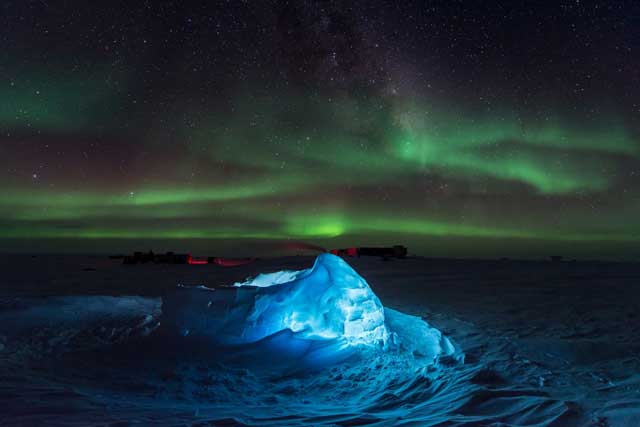A captivating and dramatic nighttime photograph showcasing the mesmerizing Northern Lights, or Aurora Borealis, illuminates the top two-thirds of the frame with vibrant green, curtain-like patterns and a scattering of stars against a backdrop of dark clouds. In the foreground, a peculiar, roofless igloo glows blue from internal lighting, its walls casting a serene hue across the surrounding snow. Just below the horizon, the partially lit ocean reveals waves and possibly an iceberg or a large ice flow, bathed in light and appearing to drift rightward. The horizon features indistinct dark structures, potentially ships or buildings, marked with red lights—adding to the enigmatic allure of this visually stunning scene.